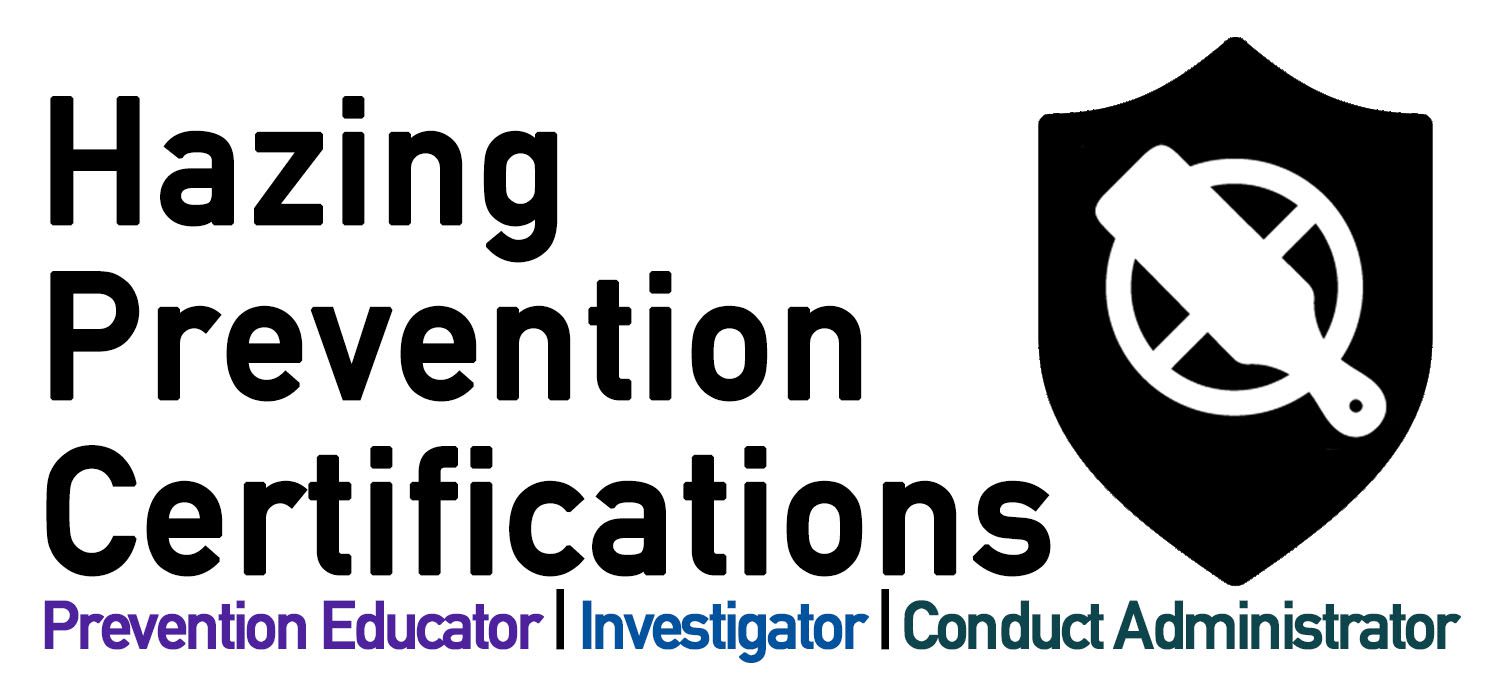The image features an advertisement aimed at deterring college hazing. On the right side, a black, medieval-style shield displays a white circle with a diagonal line, symbolizing prohibition. Within this circle, there's a white paddle, typically associated with hazing, indicating it's forbidden. On the left side, the black text reads "Hazing Prevention Certifications." Below it, in purple, it says "Prevention Educator," followed by a vertical black line, then in blue, it says "Investigator," followed by another vertical black line, and finally, it says "Conduct Administrator" in dark green. The shield and paddle imagery reinforce the message against hazing, with the various titles suggesting roles certified to prevent it.